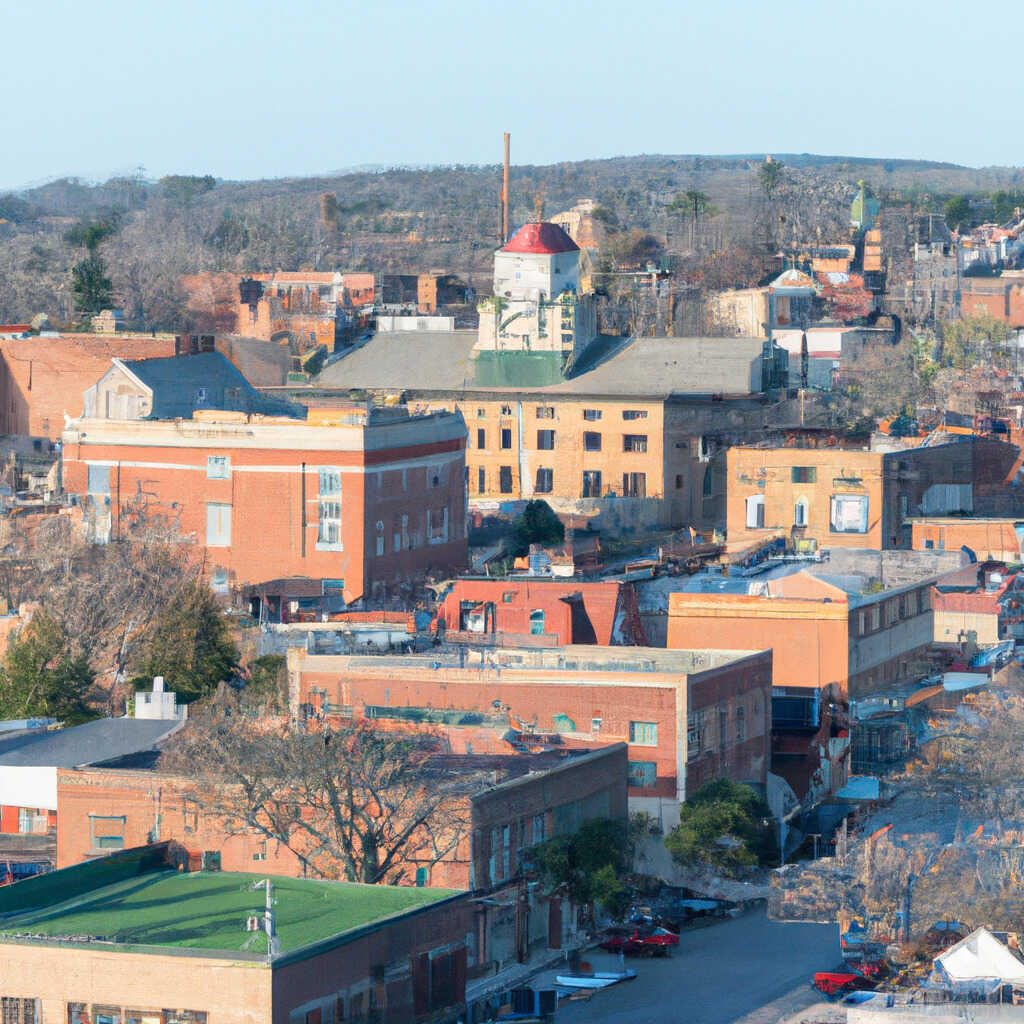This is an overhead shot of a small factory town, dominated by a mix of old brick buildings in shades of brown, gray, and red. Many of the structures are two to four stories high, and one prominent building in the center has a green roof and features a unique tower with a green cloth, a white middle section, and a red domed top with an object protruding from it. Surrounding the buildings are scattered green trees and some dead trees, with mountain hills visible in the background. The image also shows blue skies above, adding a touch of brightness. In the foreground, there's a street lined with various metal objects, scaffolding, and a few parked red cars, giving a somewhat abandoned appearance. Additionally, there are power lines running across the top portion of the image.